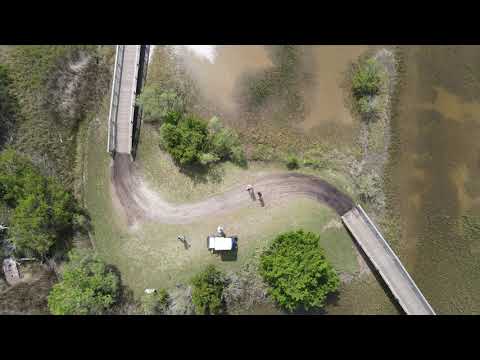In this detailed aerial view of a countryside scene, a winding, S-shaped gray paved road starts from the bottom right corner, snaking through patches of green grass and clusters of lush trees. The road crosses a gray wooden bridge with railings, continuing vertically until it disappears at the top of the image. Two individuals are seen walking at the center along the road, with a white-roofed car parked just below them and surrounded by several trees. Towards the left, there's a small building nestled amongst more trees. Above this central section, further up the road, lies the continuation of the bridge while a little to the right, there's a noticeable area of brown dirt. Water bodies flank the scene, with one visible in the top right and another sandy, water-edged area on the bottom right, adding to the serene, natural setting.